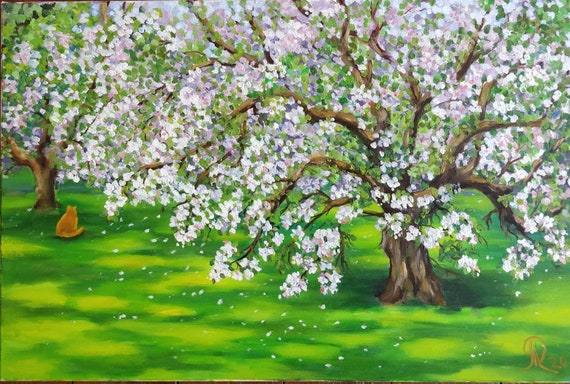This rectangular artwork, approximately four inches wide and two to three inches high, portrays a dreamy, surreal scene created with either oil paint or AI, though the low-resolution image makes finer details hard to discern. The painting features a large tree on the right and a smaller one on the left, both adorned with abundant cherry blossoms in shades of white, pink, and purple. The blossoms extend from thick brown trunks and long branches, creating an enchanting canopy. Below the trees, an orange cat faces away from the viewer, nestled amidst deep green grass, which is highlighted with vivid, irregular-toned patches of light yellowish-green to depict sunlight filtering through the foliage. The bottom and left edges of the image are bordered by a thin, brown line that extends slightly over to the right at the top. In the lower right-hand corner, the artist’s signature is displayed in gold paint, resembling a capital M over an R, with "ZO" next to it. Scattered flower petals add a whimsical touch to the lush grass below, enhancing the painting's ethereal quality.